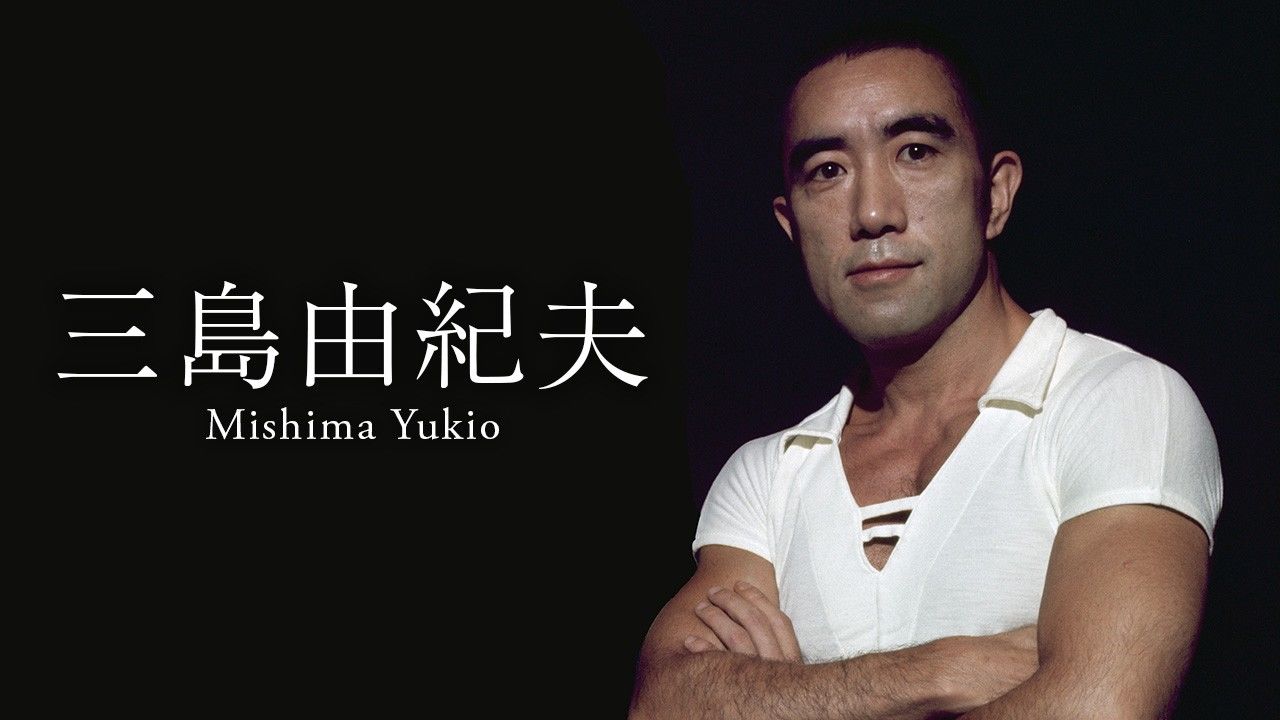The image features a striking poster set against a deep black background. Central to the composition is a portrait of an Asian man with short black hair, heavy black eyebrows, and dark, intense eyes. He is dressed in a short-sleeved white shirt, standing confidently with his arms crossed. His expression is determined and serious, yet not unkind—capturing a sense of resolve without appearing overtly stern. To the left of his image, large Chinese characters are prominently displayed in bold strokes. Below these characters, in stark white lettering, the name "Mishima Yukio" is elegantly written. The overall mood of the poster is intense yet captivating, commanding attention and respect.